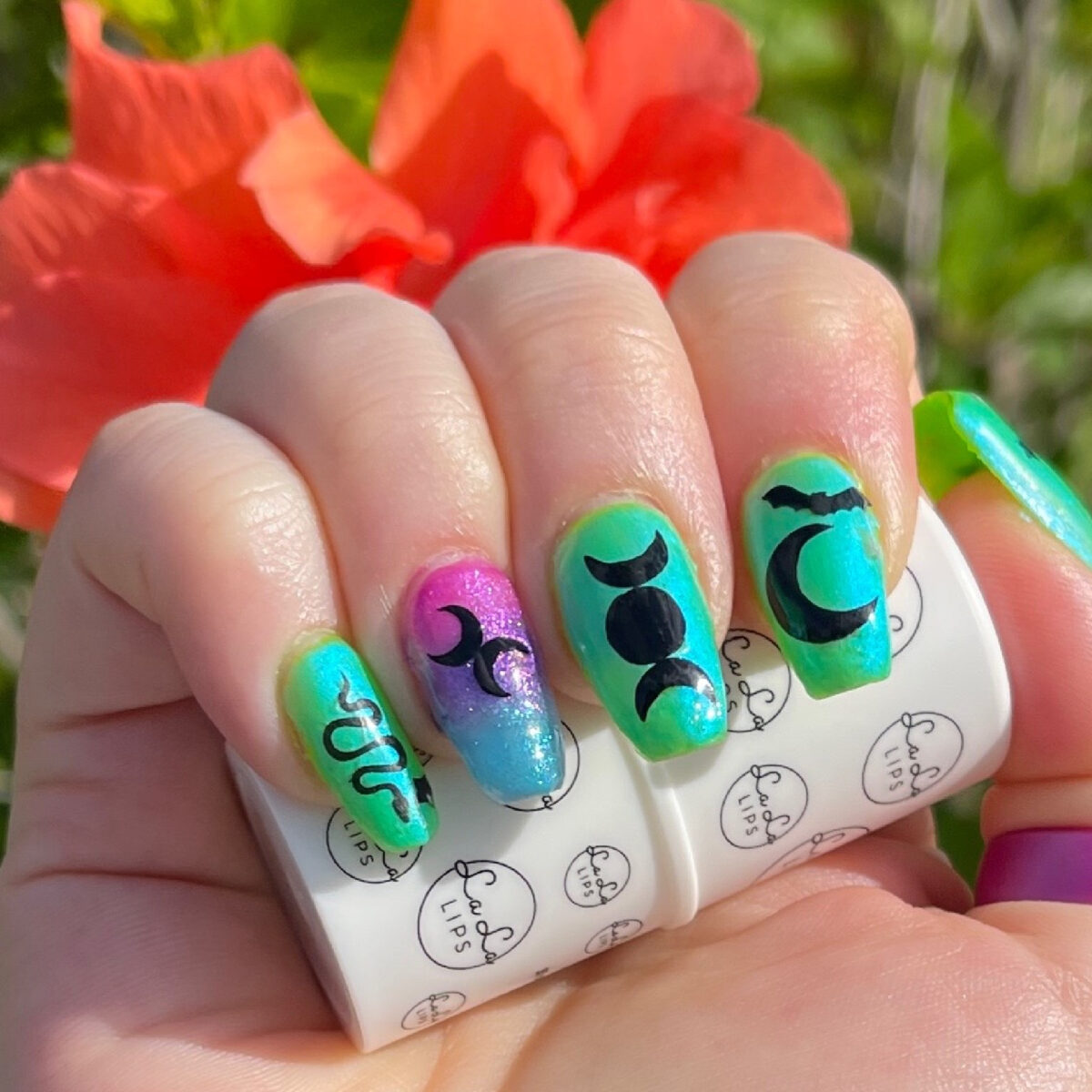The image showcases a woman's hand, adorned with vividly painted nails, gripping a white cylindrical container labeled "La La Lips" in black text and circular design. The fingernails display a variety of designs: the pinky nail is bright green with a black snake; the ring finger transitions from pink to purple to blue with two silver moons side by side; the middle finger is bright green with a circular design featuring silver moons; and the index finger, also bright green, displays a silver moon and a black bat. Her thumb, positioned to the right, features a long green nail with intricate imagery and is accessorized with a purple thumb ring. The background is artistically blurred, focusing on a vibrant orange poppy flower against lush green foliage, enhancing the hand's bright white skin and the intricate, goth-themed nail art.